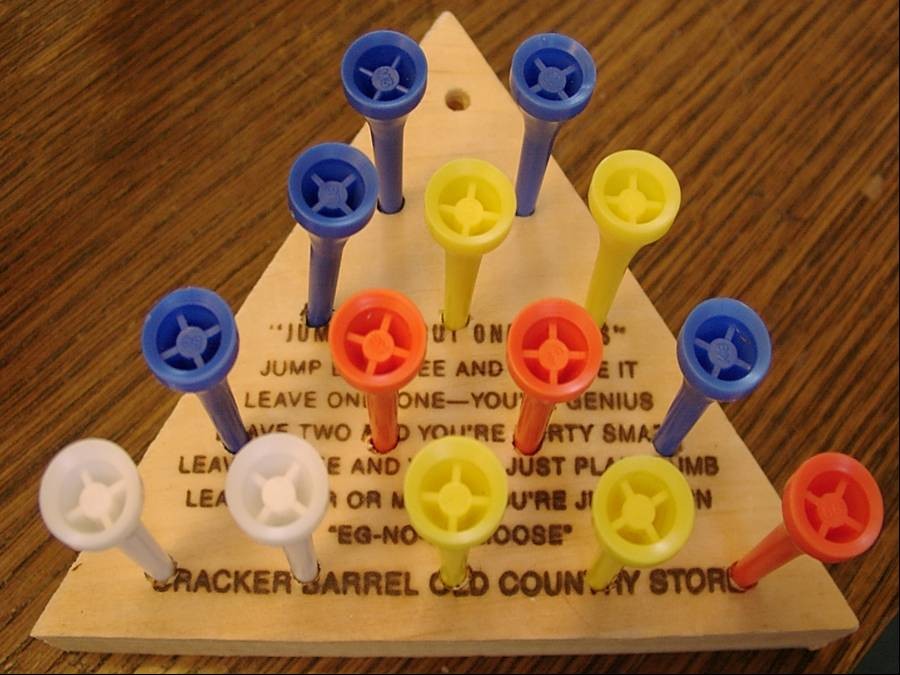This detailed photograph showcases a kid's toy that doubles as a handheld wooden game, commonly found at Cracker Barrel Old Country Store. The game features a triangular base made of light brown wood with darker brown engraved text. While most of the text is obscured by the pegs, the visible line at the base reads "Cracker Barrel Old Country Store" and appears to contain instructions on how to play.

The wooden triangle has a total of 15 holes, hosting 14 plastic pegs in various colors: blue, yellow, orange, red, and white. The pegs are meticulously arranged in ascending rows from the base to the tip of the triangle as follows:

- **Base row:** White, white, yellow, yellow, red
- **Second row:** Blue, orange, orange, blue
- **Third row:** Blue, yellow, yellow
- **Fourth row:** Blue, blue
- **Top row:** One empty hole at the tip

The distribution of colors includes five blue pegs, four yellow pegs, three red pegs, and two white pegs. Each peg is snugly fitted into its respective hole except for the solitary top hole, which is left vacant, inviting players to engage in the game's intriguing challenge.